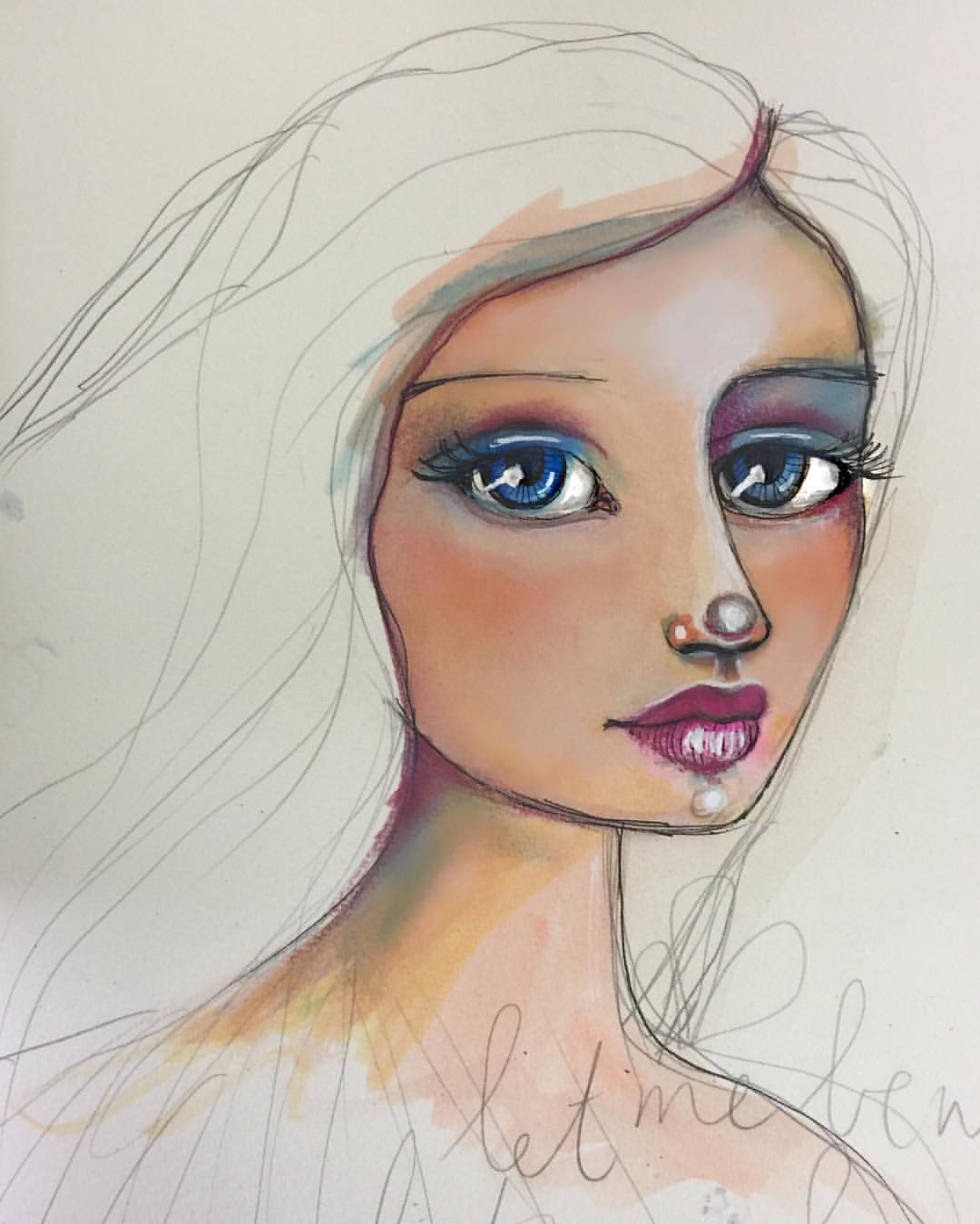A captivating sketch-painting features a young girl, her expressive face and neck meticulously painted while the rest of her body remains in pencil. Her intriguing blue eyes seem to hold shadows, giving them an almost haunting depth. She wears a shade of red, almost pink, lipstick, and has a subtle application of eye shadow around her eyes. A touch of pink is subtly visible at the back of her neck, but the natural skin tones are limited to her face and neck. Notably, there is a peculiar grayish-white lump at the tip of her nose, accompanied by a small white hole on the side, contrasting against a darker orange background. In the bottom right corner of the sketch, the phrase "Let me be" is scribbled, adding an element of melancholy to the artwork.